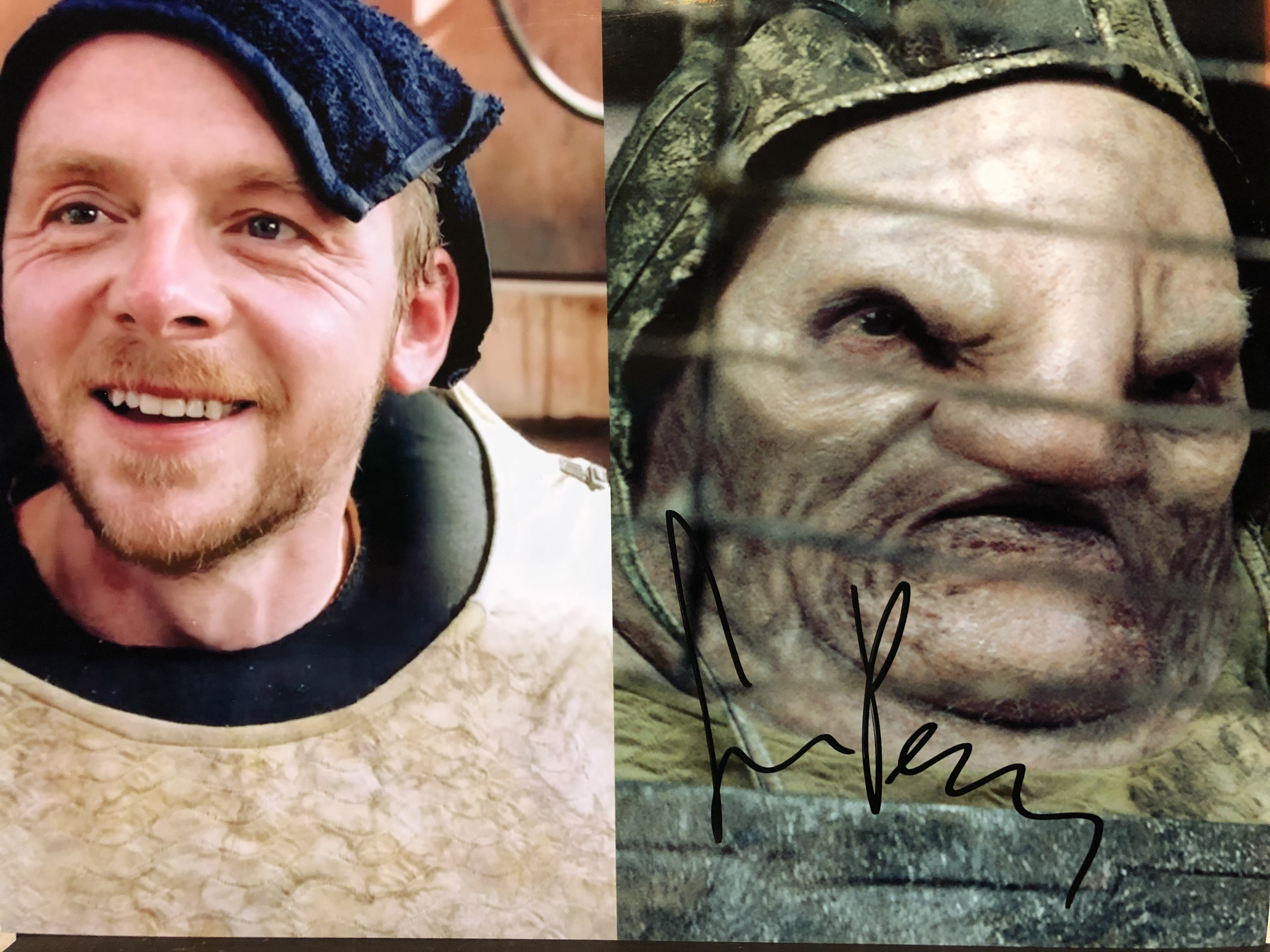This image showcases two distinct figures side by side, likely from a movie production. On the left, a smiling English actor, known for his lead role in "Shaun of the Dead," is captured during a dressing room preparation. He sports a navy blue washcloth on his head and has a short beard. His costume includes a padded collar around his neck and a sheet draping over his lower body. On the right side, the image features a ghastly, monstrous character with a swollen face, large nose, and an expression of disgust and anger. The monster appears to have some form of headgear and a metal chest plate as part of its costume. An autograph is visible over the monster's image, implying a connection between the actor on the left and the character on the right, showcasing the transformation from actor to fully costumed monster.